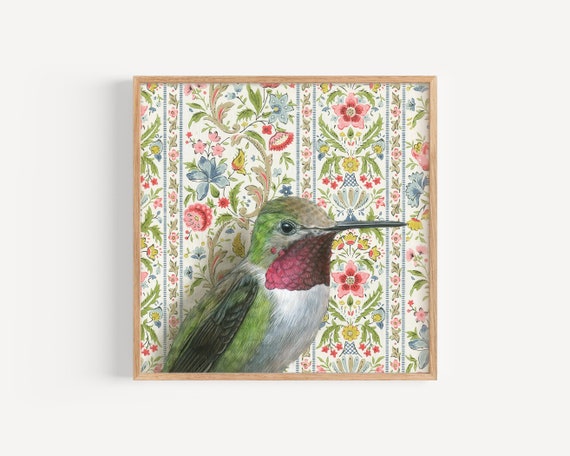The image depicts a striking ruby-throated hummingbird with a green head and body adorned with light and dark green feathers. Its throat features a vibrant ruby-red patch, contrasted by a cream-colored chest below. The bird’s long, sharp, slightly gray beak adds to its detailed elegance. Set against an intricate floral wallpaper, the background showcases a delightful medley of pink, blue, and yellow flowers interspersed with green leaves and light blue vertical cross lines. This wallpaper is framed by a light tan or wooden border, beautifully complementing the hummingbird's vivid colors and giving the entire composition a visually pleasing, painterly quality. The bird’s pose and expression convey a sense of satisfaction, adding a touch of personality to the overall scene.